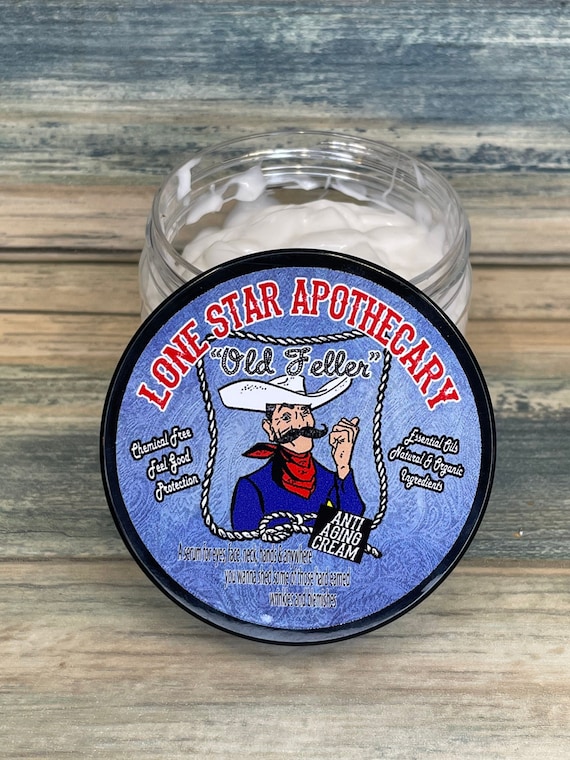The image captures a close-up, top-down view of a wooden picnic-type tabletop made of horizontal planks in hues of brown and gray. Centered on the table is a small, shallow, clear glass jar containing a white cream or liquid. The jar's lid is propped up against it, revealing a detailed label. The circular lid features a black rim and a blue background that resembles denim. The label on the lid prominently reads "Lone Star Apothecary" in red lettering with a white border. Below the text is an illustration of a cartoon gentleman within a lasso frame, who wears a blue long-sleeve shirt, red bandana, and white cowboy hat. The man's mustache curls up on each side. Surrounding the illustration, the text reads "Old Feller" and "Chemical Free, Feel Good, Protection, Anti-Aging Cream."